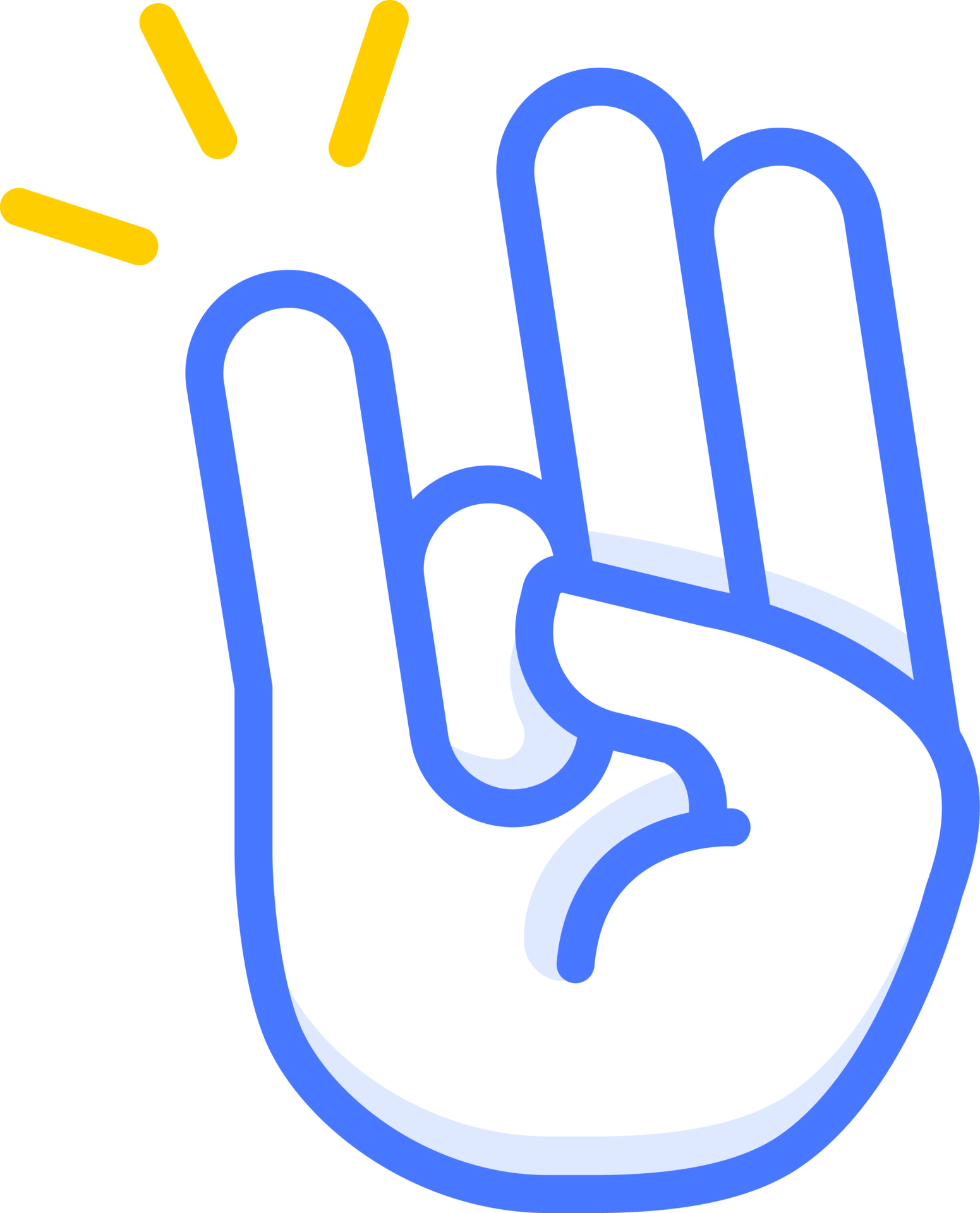The image depicts a blue, cartoon-like outline of a right hand with the pointer, middle, and pinky fingers extended upwards, while the thumb and ring finger are bent down towards the palm, with the thumb touching the ring finger. Above the pinky finger, there are three golden-yellow lines suggesting a snapping effect or action. The image appears as a symbol or logo and is known as "the shocker." The hand has no additional coloring or details such as nails, giving it a simplistic, emblematic look.